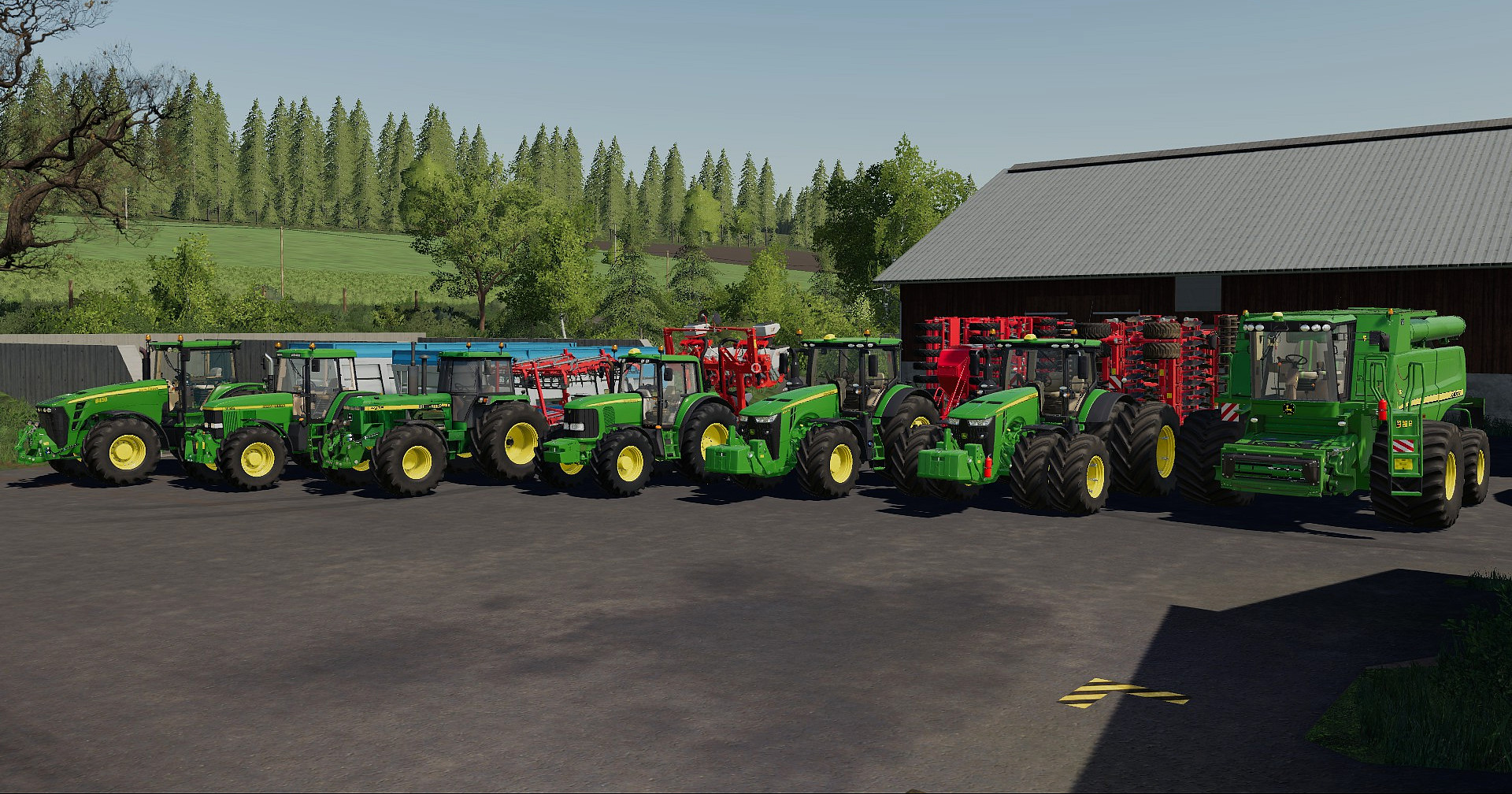The image depicts a large lot populated with green tractors, each featuring yellow wheels and a yellow stripe on top. The tractors are neatly parked in front of a brown house with a gray, slanted roof and are situated on a pavement with visible markings. Behind these tractors, there's an assortment of red farming machinery and trucks. The scene also includes another green farming vehicle on the right side. Surrounding the lot are a variety of trees, including pine and evergreen types, as well as a barren brown tree with broken branches. In the background, we can see expansive green farmlands under a vast, light blue sky. Additionally, there is a structure with a turquoise roof visible in the image. No people are present in the photograph.